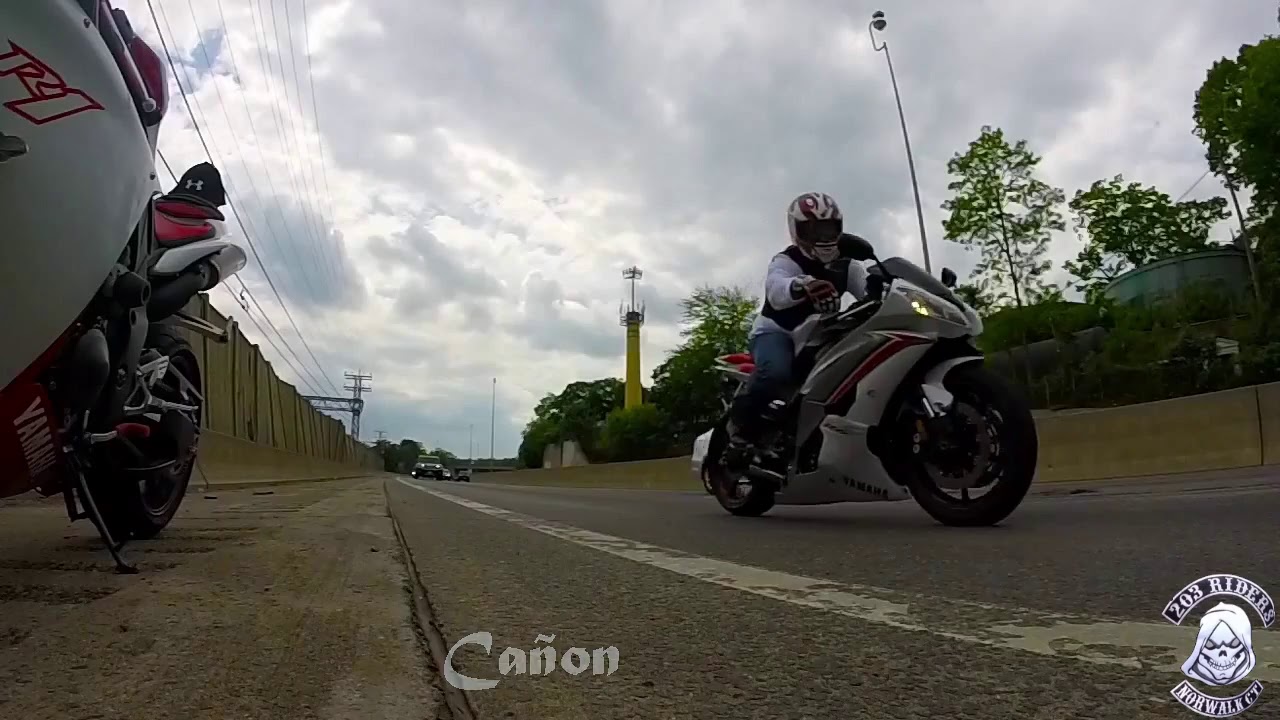The photograph depicts an outdoor scene during the daytime, focusing on a road with various elements of interest. To the left, a white Yamaha motorcycle with red, black, and gray accents is parked on its kickstand on the sidewalk. Moving towards the center-right of the image, another white Yamaha motorcycle ridden by a person in a white and red helmet, black and white jacket, and blue jeans, rides down the highway. Behind this motorcyclist, several vehicles follow on the road. In the background, there is a concrete barrier wall, some homes or possibly a low water tower, and trees. Above them, a cloudy sky with patches of blue is visible. At the bottom center of the image, the text "Cañon" is displayed in transparent white print, with a tilde over the "n." Additionally, the bottom right corner features the text "203 Riders, Norwalk, Connecticut" along with an illustration of a skull with a cowl. The color palette includes white, gray, blue, black, red, green, and yellow, and the entire setting appears to be an outdoor highway scene captured from the perspective of a bike on the side of the road.